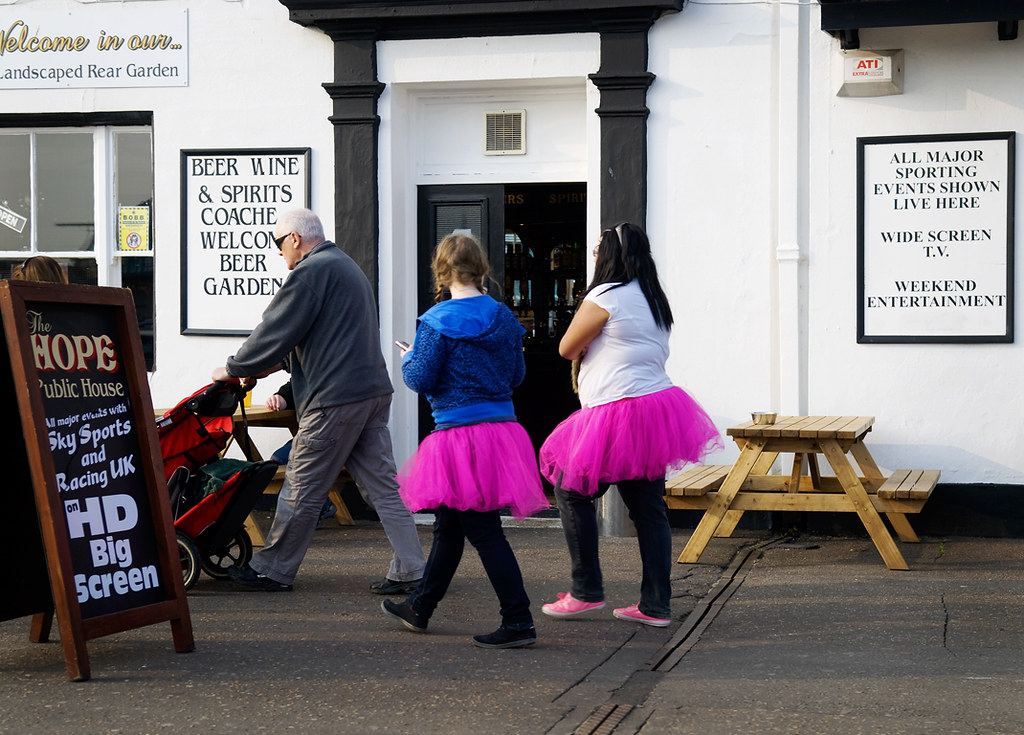In the photograph, a bright, clear sunny day illuminates an outdoor scene in front of a white building with black-trimmed windows, doors, and pillars. Dominating the scene is an elderly man with short gray hair, dressed in a gray sweater and pants, wearing dark sunglasses. He is pushing a red and black baby stroller. Walking behind him are two younger women in bright fluorescent pink tutus and black pants. One of the women has long blonde hair and is wearing a white shirt, while the other has long dark hair and wears a blue hoodie. They are facing the building, making their faces not visible.

The building has several prominent signs and banners. On the left wall, a sign reads "Beer, Wine, and Spirits, Coaches Welcome, Beer Garden." To the right, another sign states "All Major Sporting Events Shown Live Here, Widescreen TV, Weekend Entertainment." Below these signs, further details are displayed on a sandwich board that reads "The Hope Public House, All Major Events with Sky Sports and Racing UK HD on Big Screen."

In front of the building, two picnic tables are positioned, with one on the right being unoccupied. The table on the left, slightly harder to discern, has a person sitting at it with a tall beer in front of them. The overall atmosphere is lively and inviting, giving a sense of community and leisure.